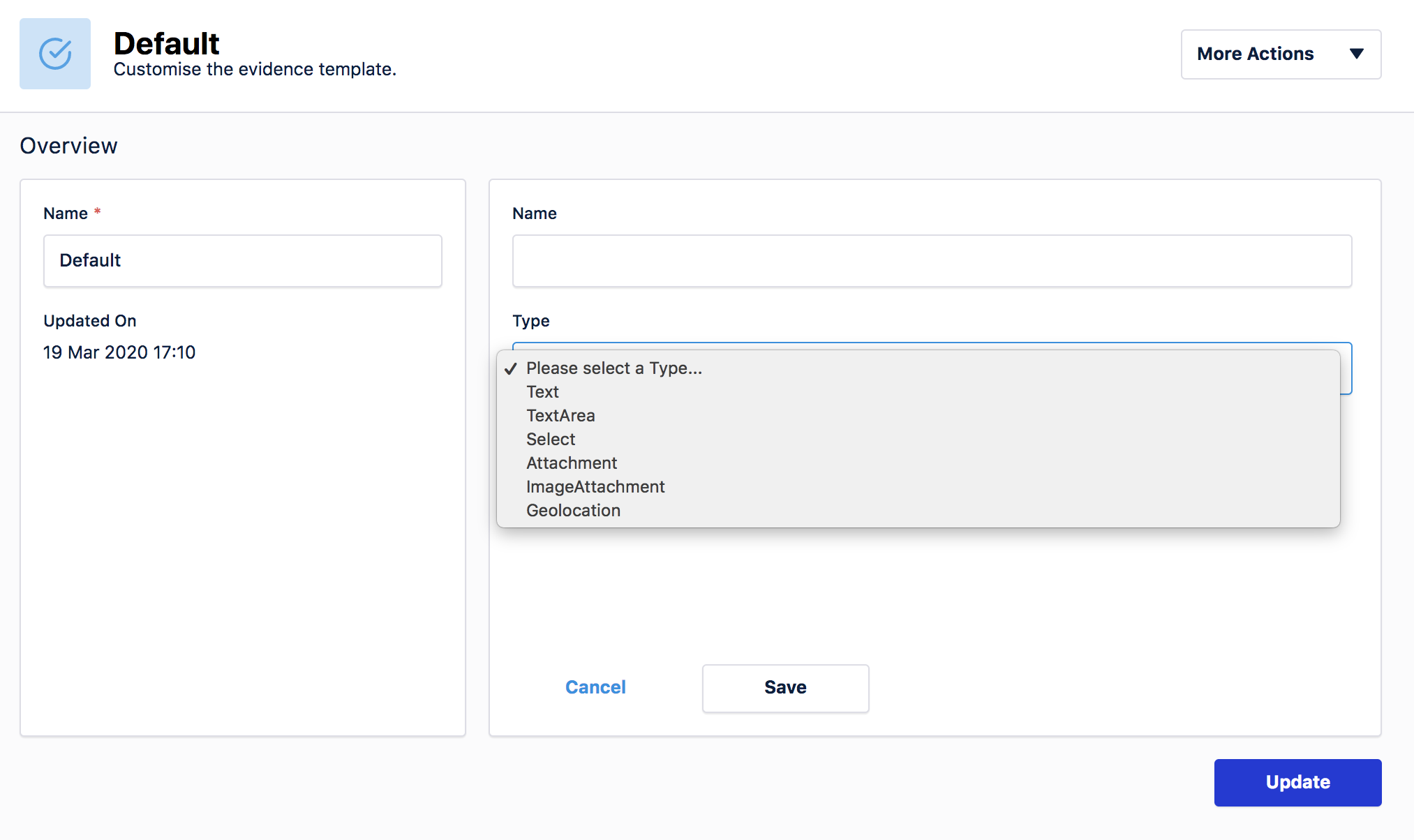This image is a screenshot primarily displayed against a white background. In the upper left corner, there is black bold text adjacent to a light blue square containing a checkmark, reading "Default - Customize the evidence template." On the upper right side, within a white box, there is an option labeled "More actions."

Below this, a light gray horizontal line spans the width of the screenshot. Underneath the line, on the left side, the section is titled "Overview." Directly below "Overview," enclosed within a small box, there is text indicating "Name: Default," followed by "Updated on: 19 Mar 2020 17:10."

To the right of this section, there is another light gray box. Inside this box, there are labeled fields for "Name" with a corresponding input field below it. Following the "Name" field, there is another label "Type," with a dropdown menu offering various options such as "Please select a type," "Text," "Text area," "Select," "Attachment," "Image attachment," and "Geolocation."